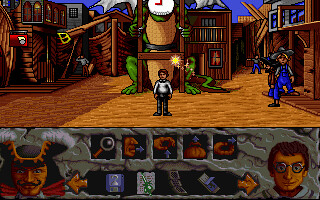In this pixelated, retro-style video game screenshot, the upper half of the image features a majestic dragon encased in a wooden frame, giving the appearance of it being boxed. The scene is set in the heart of a quaint, bustling town constructed entirely of boats. In the center stands a character in a white jacket and grey pants, notably adorned with a pair of Beats by Dre headphones around his neck. To the right, a hillbilly character donning blue coveralls and a grey cowboy hat can be seen, with another figure in blue jeans, a brown shirt, and a dark hat positioned in front of him. The bottom of the image showcases a pirate to the left and a Harry Potter look-alike to the right. Centrally placed are various interactive symbols, including a bag, pairs of hands, a single hand, a mouth, a turd, and a magnifying glass, indicating different actions available to the player.